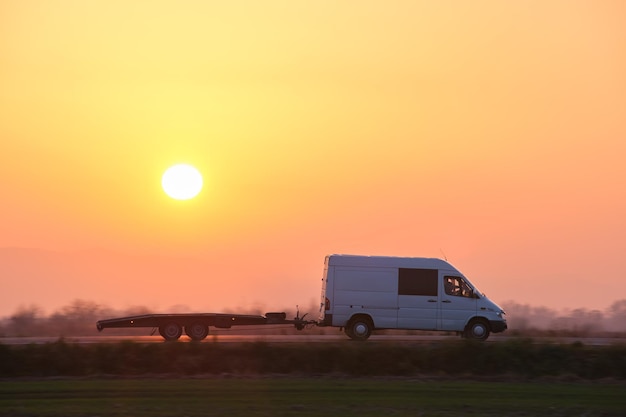In the vibrant scene, a white, two-door cargo van, identifiable by its slanted front window and squared-off back, travels along a road with a flatbed trailer in tow. The front of the van is facing right, and the trailer, which has two closely spaced set of wheels, is empty. The road and surrounding area are shrouded in the encroaching darkness of dusk, as the bright yellow sun sits in a predominantly yellow sky that gradually shifts through orange and pink hues as it nears the horizon. This sunset sky takes up a significant portion – about 70% – of the image's frame. Below the sky, a blurred tree line stretches along the horizon, devoid of foliage and silhouetted against the dimming light. There is also a neatly trimmed field of green grass on either side of the road, dotted with plants. While the silhouette of trees and the empty landscape dominate the lower part of the image, the setting sun enhances the scene's dramatic lighting, casting deep shadows and illuminating the colors of the sky with a radiant glow.